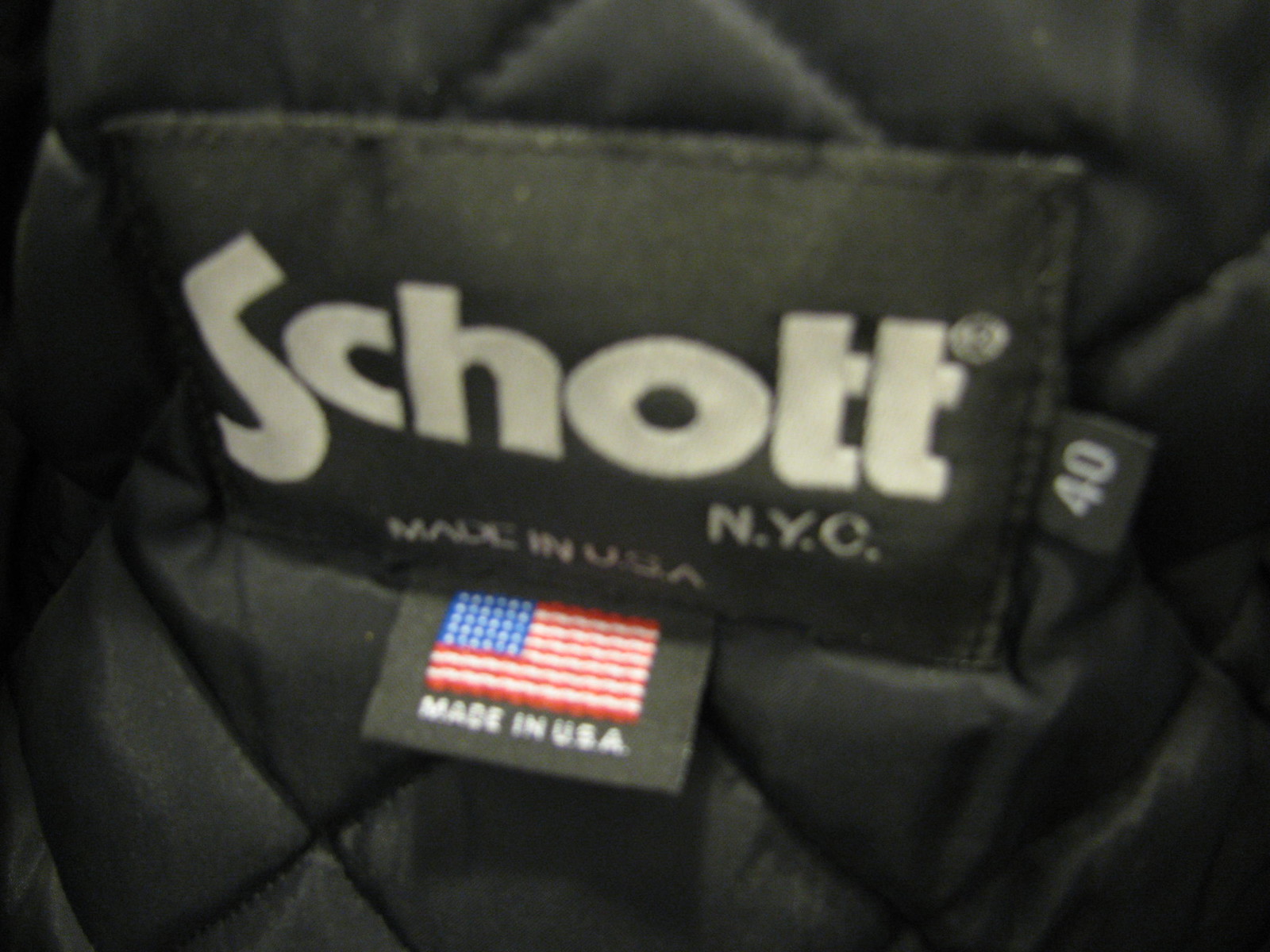The image is an extreme close-up of a section of a black jacket, showcasing three distinct fabric labels. The main label reads "SCHOTT NYC" in white text, with "Made in USA" written below it. This primary label is made of black fabric. Directly beneath it, a smaller rectangular label features an American flag, also with "Made in USA" written in white letters. To the right of these labels, there's a tiny black tab that simply bears the number "40" in white, indicating the jacket's size. The surrounding fabric of the jacket appears to be quilted in an interlocking diamond pattern, suggesting a thick, possibly quilted texture.